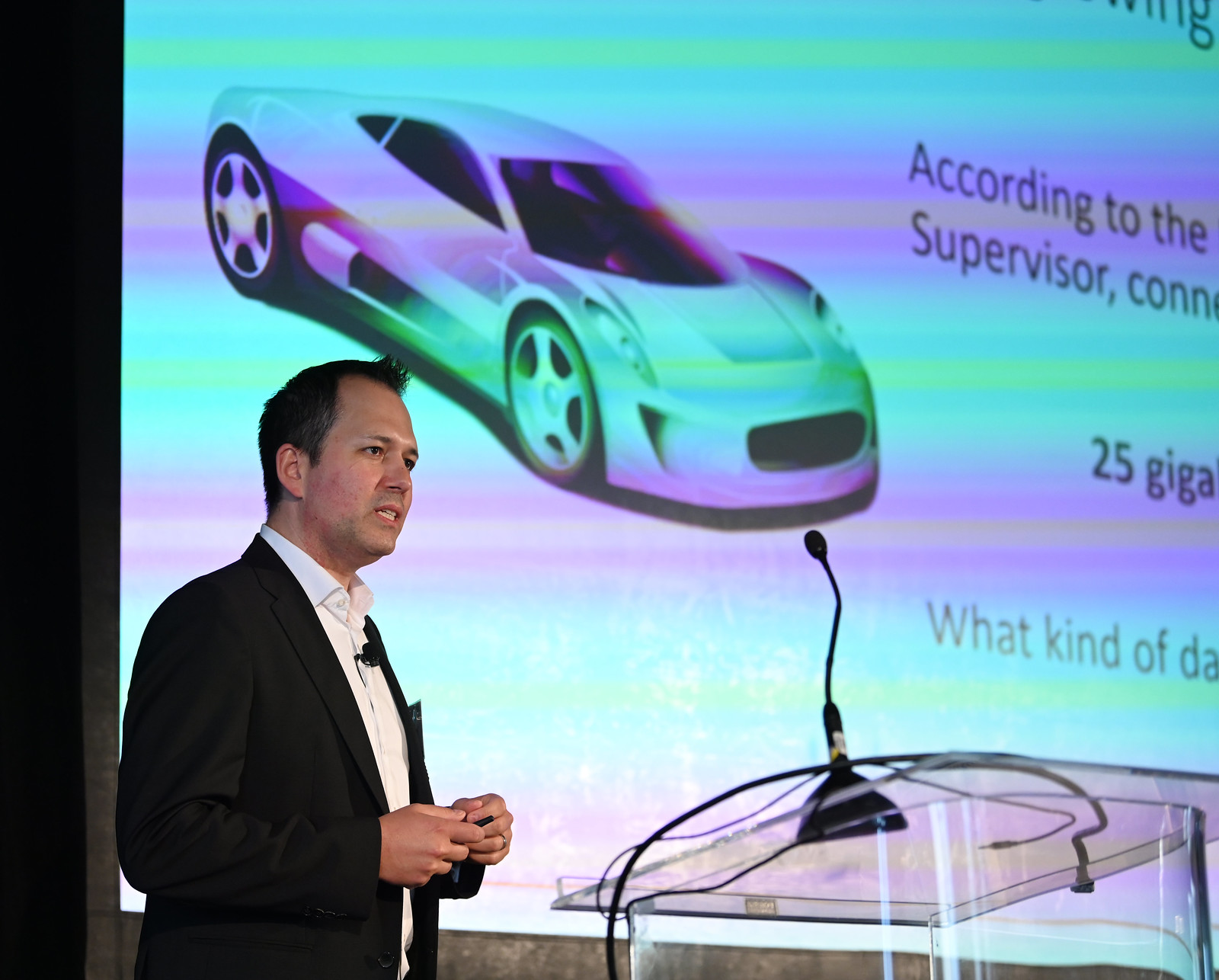The horizontal rectangular image depicts a man giving a presentation about a futuristic sports car. Standing at a clear glass podium at the front, the man is dressed in a black suit jacket, a crisp white shirt, and has a microphone clipped to the neck of his shirt. He is clean-shaven, with short, dark hair styled into a subtle mohawk. The scene captures him speaking, with a colorful projected image of a sleek, fast car above his head on a large white screen behind him. The screen, which has a slight rainbow glare effect, also shows some text cut off at the edges, hinting at technical details about the car with fragments like "according to the," "supervisor," "22 giga," and "what kind of DA." The overall setting hints at a formal event or a conference where the man is presenting what appears to be an innovative vehicle design.